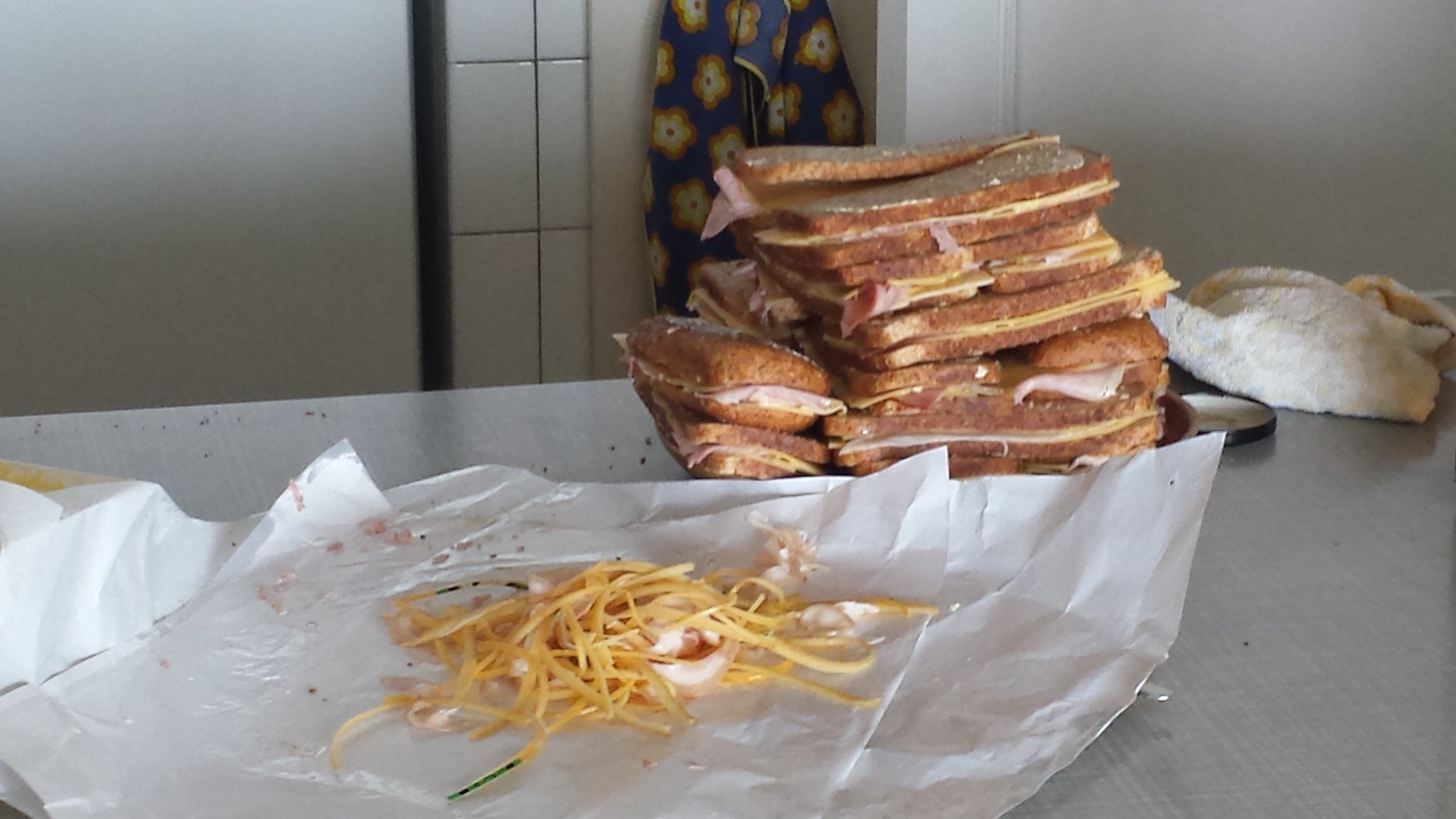This image captures a close-up scene on a gray kitchen countertop, where a neat stack of eight or more ham and cheese sandwiches sits prominently. The sandwiches, varying in bread color between dark brown and white, are made with slices of white bread, some using the heel slices. Positioned to the left, there's parchment paper with what appears to be shredded yellow cheese, suggesting some of the cheese was removed from the sandwiches and left in the wrapping. To the right of the sandwiches, a cream-colored towel is laid out on the counter. In the background, a white tiled wall can be seen partially, along with a dark blue apron adorned with white flowers outlined in yellow, hanging against the white walls. The photo is closely focused on the sandwiches, making the finer background details slightly blurred but identifiable.